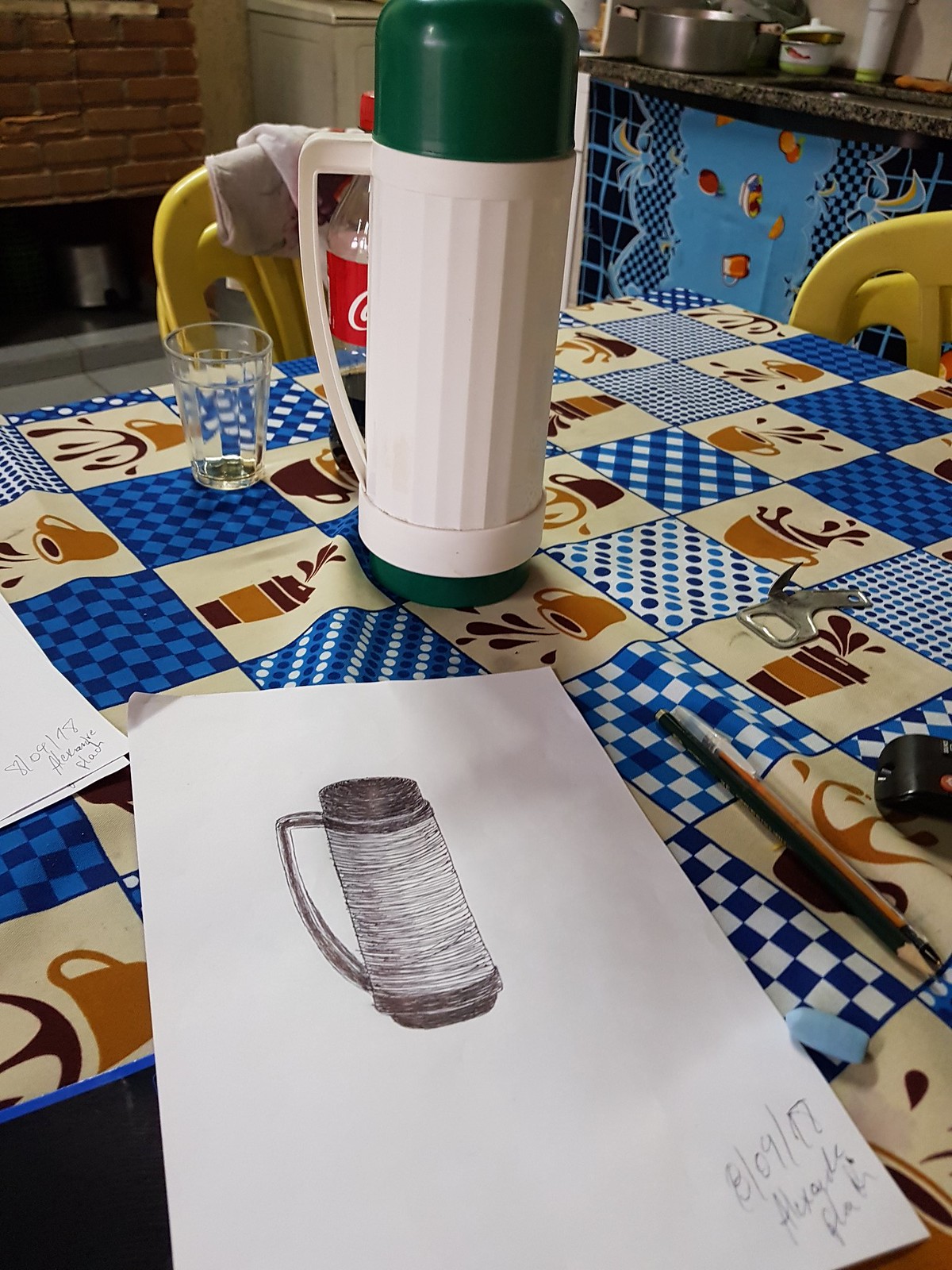A detailed image captures a scene in what appears to be a kitchen. Central to the composition is a white plastic flask with a green lid, prominently placed on a tabletop surface, which may be covered with a cloth. The background reveals a kitchen sink with a metal dish resting beside it, and in the top left corner, there is a glimpse of what might be a fireplace. Surrounding the table are yellow plastic chairs adding a pop of color to the scene. On the same table, a sheet of paper displays an artistic sketch of the flask. While the sketch is drawn in monochrome and somewhat simplifies the flask's design, it approximates the general shape and includes the handle. Notably, the green lid and the vertical lines of the actual flask are absent in the drawing, suggesting the artist may have sketched it when the lid was not in place. This juxtaposition of the real flask and its imperfectly rendered counterpart adds an intriguing layer to the everyday kitchen tableau.